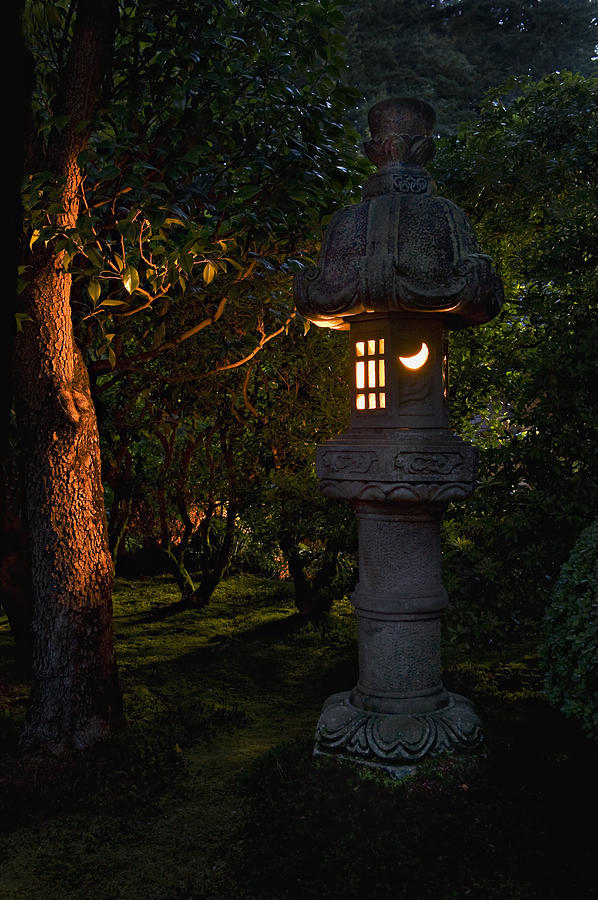In this vertical, dark, and almost fairy-tale-like photograph, we see a garden or dense forest setting. The scene is dominated by an Asian-influenced, pagoda-like statue that stands tall with a dome-like appearance and a large base. The statue features a built-in door or window, adorned with a crescent moon cut-out and nine small rectangular openings, from which a warm, yellow light emanates. This light illuminates the gnarled bark and branches of a tree positioned to the left of the statue, casting an eerie yet romantic glow. The surrounding area is filled with lush greenery and grass, revealing patches of sky indicating that it is close to sundown. The scene is primarily dark, yet the ethereal light from the statue pierces through, highlighting parts of the grove and adding a mystical quality to the image.